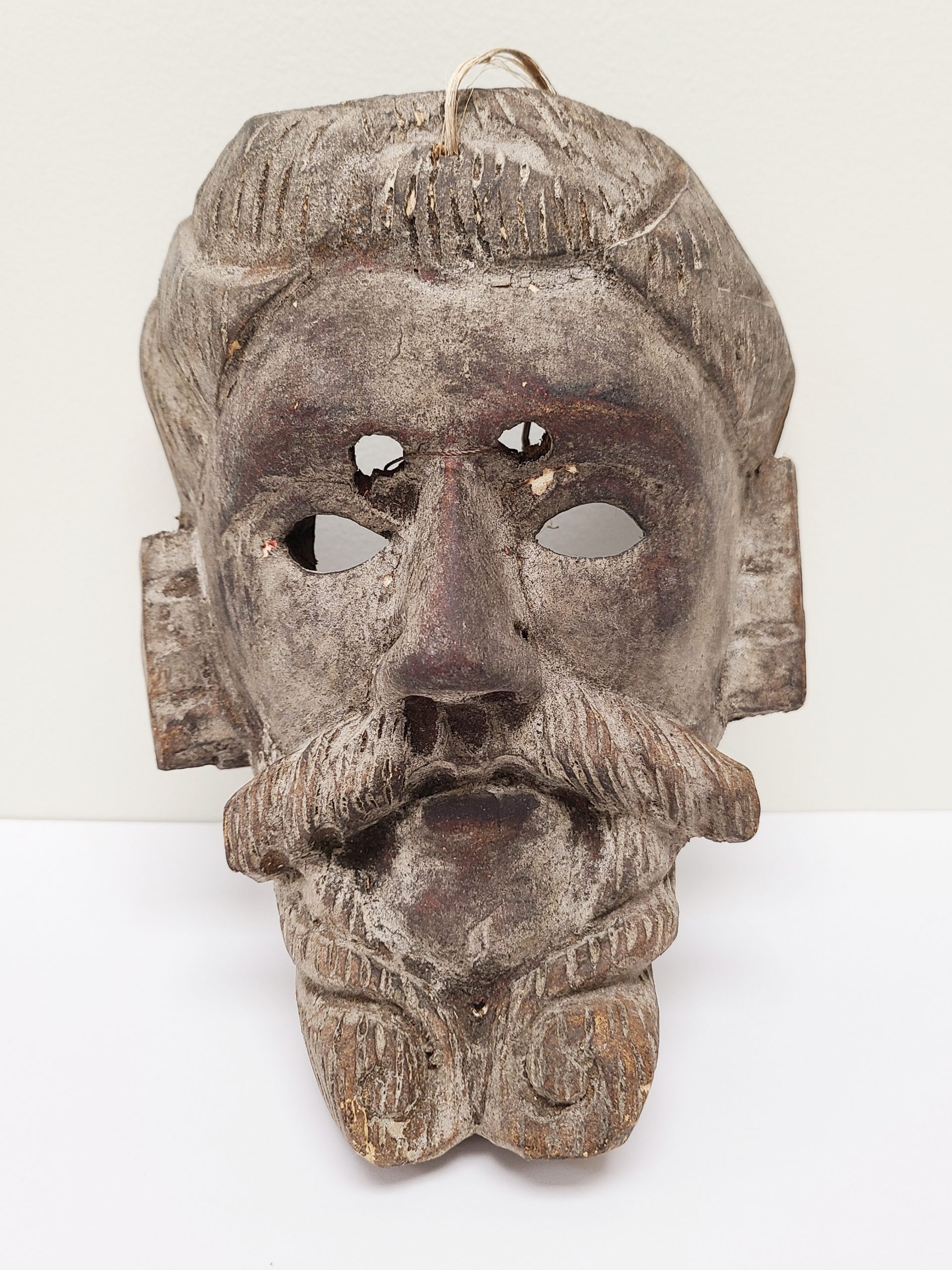The image depicts a tall rectangular background with a distinct bicolor division, where the bottom part is white and the top part is tan. Positioned against this backdrop is an ancient, weathered artifact, likely a mask or a statue, carved out of a brownish material, possibly wood or stone. The artifact represents the head of a man with pronounced features. The figure has a large, curved mustache and a detailed, ornate beard, extending outward and down, suggesting a sense of importance or nobility.

The mask's eyes are marked by deep cutouts, while two smaller holes are strategically placed above the eye openings, potentially serving as ventilation or attachment points, possibly for viewing if worn as a mask. Additionally, there are noticeable square ears and further intricate carvings denoting a serious, aged visage. There appears to be a thread or rope running through holes at the top of the head, suggesting it was once hung or possibly worn.

The craftsmanship extends to the depiction of short hair and sideburn-like features, indicative of the era and skill of the artisan. The color palette of the mask ranges from faded brown to gray, enhancing its ancient and solemn appearance. This relic exudes a sense of mysterious historical significance, somewhere between the realms of ancient and more recent archaeological finds.